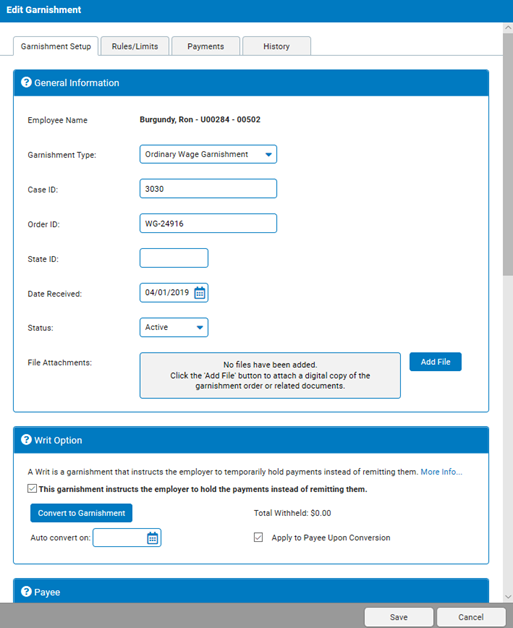Screenshot of a Website Showing Garnishment Editing for Employee Ron Burgundy

This screenshot depicts a webpage where the user has navigated to the garnishment editing section. The employee in question is Ron Burgundy, identifiable by his employee ID. The user has selected the "Ordinary Wage Garnishment" option, with a case ID of 3030 and an order ID of WG24916. The date received is recorded as January 4, 2019, and the status of the garnishment is marked as "Active."

No files have been attached yet, prompting the user to click the "Add File" button to upload a digital copy of the garnishment order or related documents. There is an explanatory option under the heading "Writ," which details that a writ instructs the employer to temporarily hold payments instead of disbursing them. The user has checked the box to indicate that this garnishment instructs the employer to hold payments.

Additionally, there is an option labeled "Convert Garnishment," showing that the current withhold amount stands at zero dollars. It mentions that the withheld amount will be applied to the payee upon conversion. At the bottom of the screen, two buttons are visible for the user to either "Save" the changes or "Cancel" them.

Overall, this screenshot provides a comprehensive view of the user interface and options available for managing employee wage garnishments.